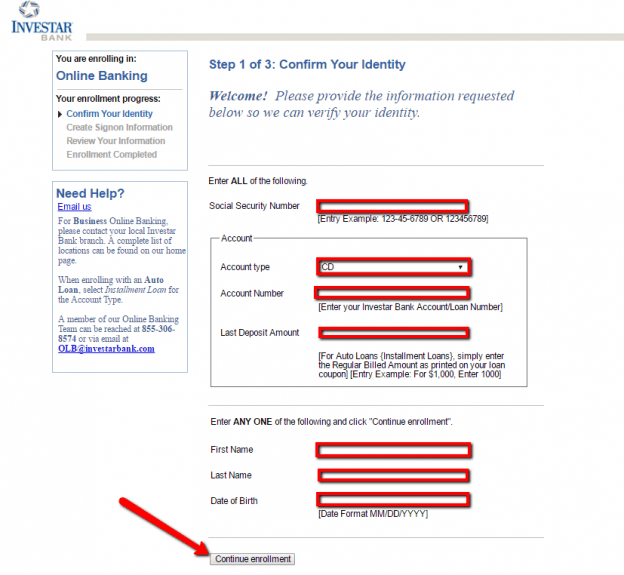Sure, here's a detailed and cleaned-up caption for the image described:

---

**Screenshot of Investar Banking Website**  

At the top of the interface, the heading "Investar Bank" is prominently displayed. To the right of this title is a gray bar. Below the heading, there's a blue header that reads "Step 103: Confirm Your Identity."

Underneath this blue header, the word "Welcome" appears in bold and italicized text. Following this, non-bold but italicized text instructs the user to "Please provide the information requested below so we can verify your identity."

There is a horizontal line separating these instructions from the next section. The next section begins with a directive in uppercase: "ENTER ALL of the following." The user is required to enter their Social Security number in the field provided, which includes an entry example and a red border around the box.

Following this, there are additional fields to be filled out, each surrounded by a red box. These fields are labeled as follows:
- "Account Type" (with a dropdown menu)
- "Account Number"
- "Last Deposit Amount"

An explanatory note is provided below these fields: "For auto loans and installment loans, simply enter the regular billed amount as printed on your loan."

Further down, another instruction reads: "Enter any ONE of the following and click Continue Enrollment." The words "ANY ONE" are in bold and uppercase. The individual fields include:
- "First Name"
- "Last Name"
- "Date of Birth" (with a reminder to enter the date in the format: two digits for month, day, and year)

A button labeled "Continue Enrollment" with a left-pointing arrow is located at the bottom of the section.

On the left-hand column, beneath the Investar Bank logo, there is a progress indicator for "Online Banking Enrollment." The current step, "Confirm Your Identity," is highlighted, and is the first of four steps. The subsequent steps listed are "Sign On," "Review," and "Enrollment Completed."

There is also a box labeled "Need Help?" with an option to email for assistance via a provided email link. 

---

This rendered caption provides a clearer, detailed explanation of the image on the described banking website.